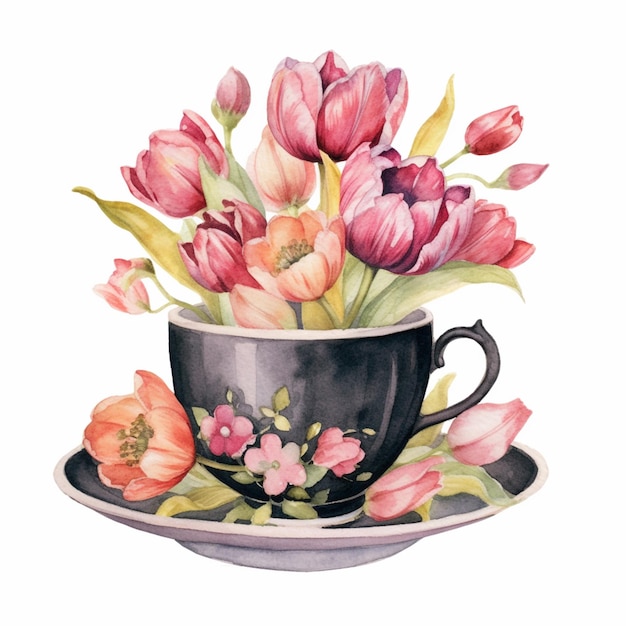This image depicts a detailed watercolor painting of a black coffee cup with a white-trimmed rim and handle, placed on a matching black saucer that features a white trim. Both the cup and saucer are adorned with an array of flowers. The saucer circles the cup with floral designs, including one open flower and two closed ones. The cup itself is filled with an abundant bouquet of flowers, predominately tulips in various shades of red, pink, orange, and light orange, alongside lush green leaves. The flowers inside the cup include an assortment of fully open blooms and two that remain closed, adding depth and diversity to the arrangement. There is also a unique floral design on the front of the cup, comprising three flowers, which enhances the overall aesthetic. The intricate details and vibrant colors of the flowers provide a striking contrast against the dark base of the teacup and saucer, making the artwork elegant and captivating.